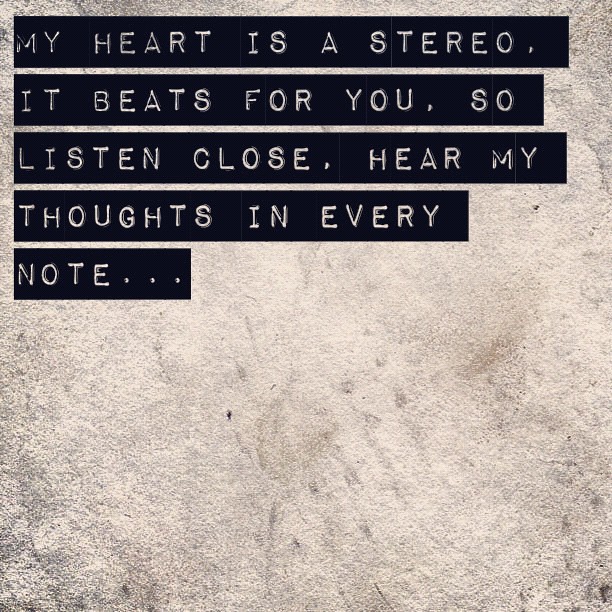The image is a vintage and rustic-themed meme typically seen on social media platforms like Facebook or Pinterest. The background mimics a grayish, distressed concrete surface, adding an edgy, worn look. Over this backdrop, there are five black strips resembling labels from a labeling gun, with white text. The text, from a song lyric by Adam Levine (also associated with Gym Class Heroes), reads: "My heart is a stereo, it beats for you. So listen close, hear my thoughts in every note...". The overall aesthetic combines a faded, tan, and silver color palette, giving the image an antiquated feel.